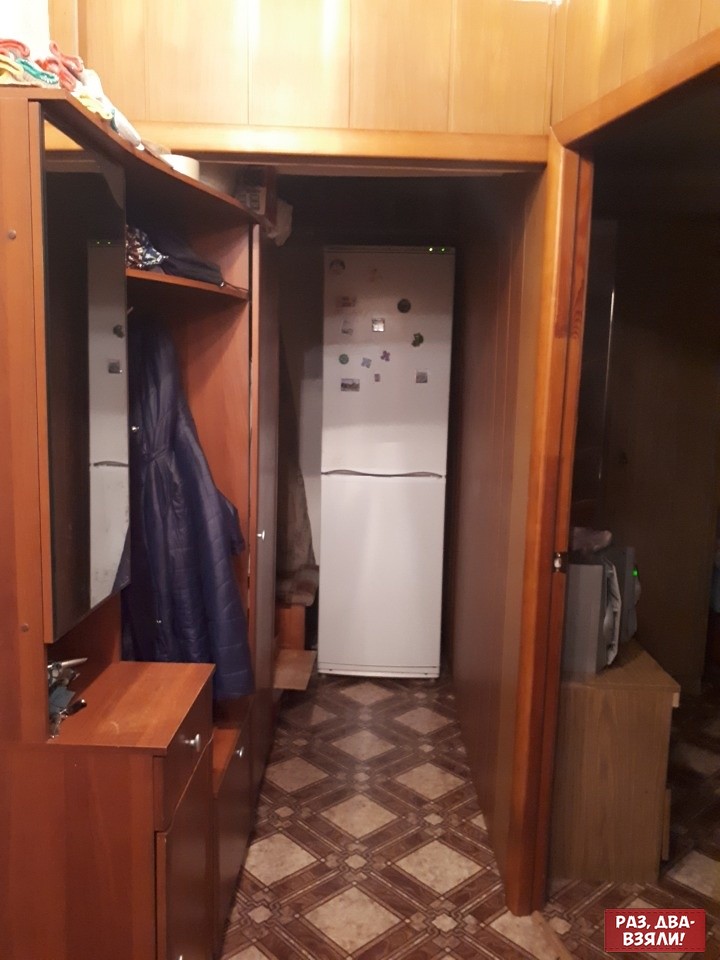This image appears to depict a small, narrow space within a house or apartment, possibly a hallway or closet area. At the center of the image, in the far back, stands a white refrigerator with a top and bottom door, adorned with several indistinguishable magnets. To the left of the refrigerator, there is a built-in cupboard space, featuring numerous drawers and some knick-knacks placed on top. A navy coat hangs from a nearby coat hanger, adding a splash of color to the scene. Above the cupboard, another storage compartment is visible, stocked with various items. On the right-hand side of the image, an open doorway leads into a darker room where a wooden dresser can be seen with what seems to be a radio or television with an antenna on top. The floor throughout this small area features a diamond pattern of tan, light tan, and slightly brown tiles. Additionally, there is a distinctive red rectangle with some text in another language, located at the bottom right-hand corner. All the walls visible in the image are wood-paneled, adding to the cozy but cramped atmosphere of the space.